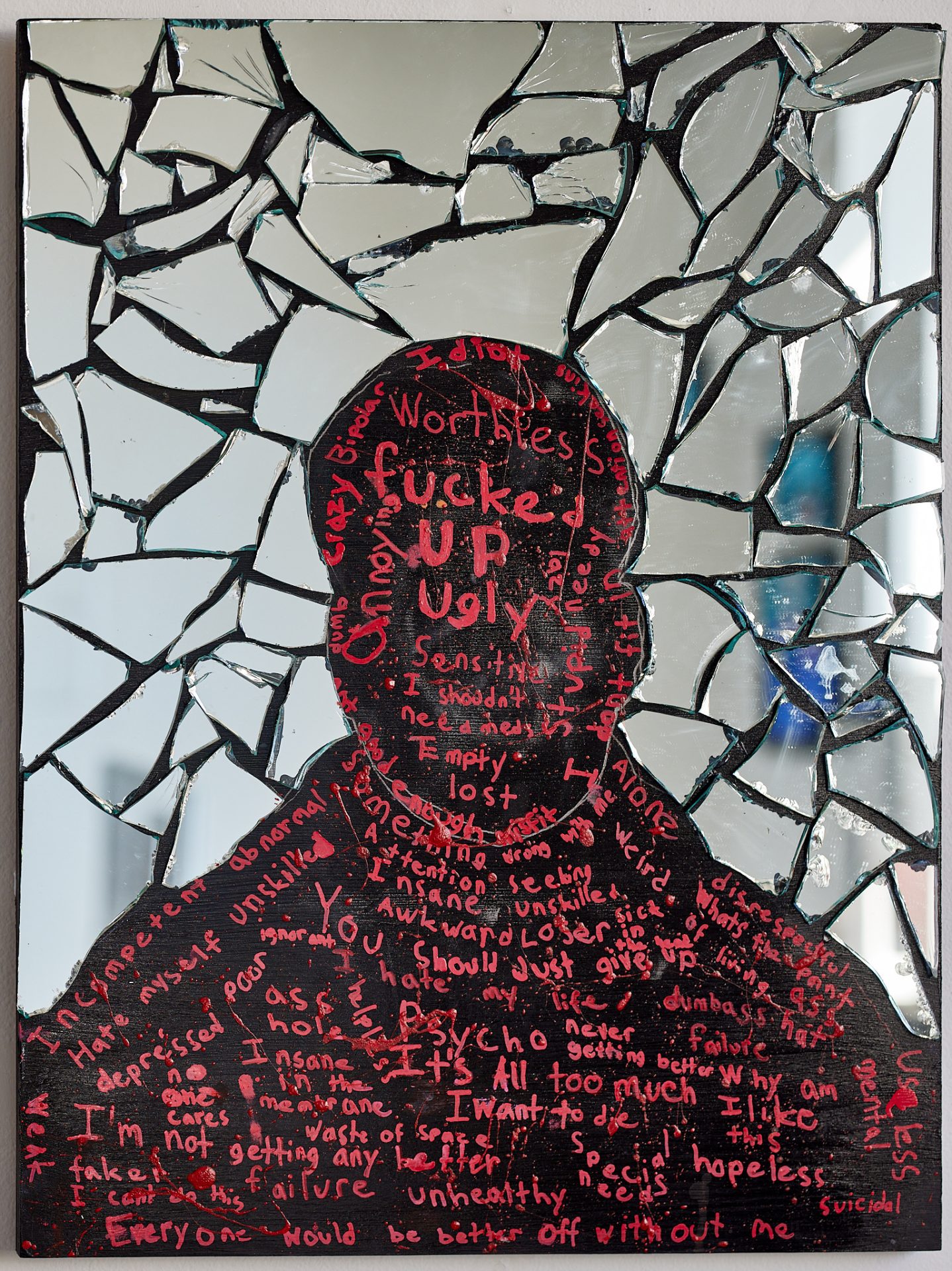This artwork, captured in a photograph, is a deeply evocative mixed-media piece combining painting and collage. At the forefront is a front-facing silhouette of a head and shoulders, vividly colored in black. This striking figure, though facing the viewer, lacks any detailed features, presenting instead a stark, hollow outline. Covering this black silhouette are numerous red inscriptions, densely packed and chaotic, bearing intensely negative words such as "worthless," "fucked up," "ugly," "empty," "lost," "insane," "awkward," "loser," amongst others. These inscriptions create a cluttered and overwhelming visual narrative of inner turmoil and self-loathing.

In the background, shattered mirror fragments have been meticulously arranged in a collage, their jagged edges forming a reflective mosaic around the figure. The broken mirror conveys a distressed and fragmented reality, with each piece reflecting fragmented and unclear portions of what appears to be a white or gray surface, interspersed with hints of blue. The black lines between the mirror pieces add to the chaos and disarray of the composition.

The overall piece evokes a powerful sense of despair, with the broken mirror symbolizing a fractured self-image and the harsh red text embodying the relentless negative thoughts that plague the figure. This poignant and dark artwork offers a raw, unsettling glimpse into the psyche of someone grappling with deep-seated emotional distress.